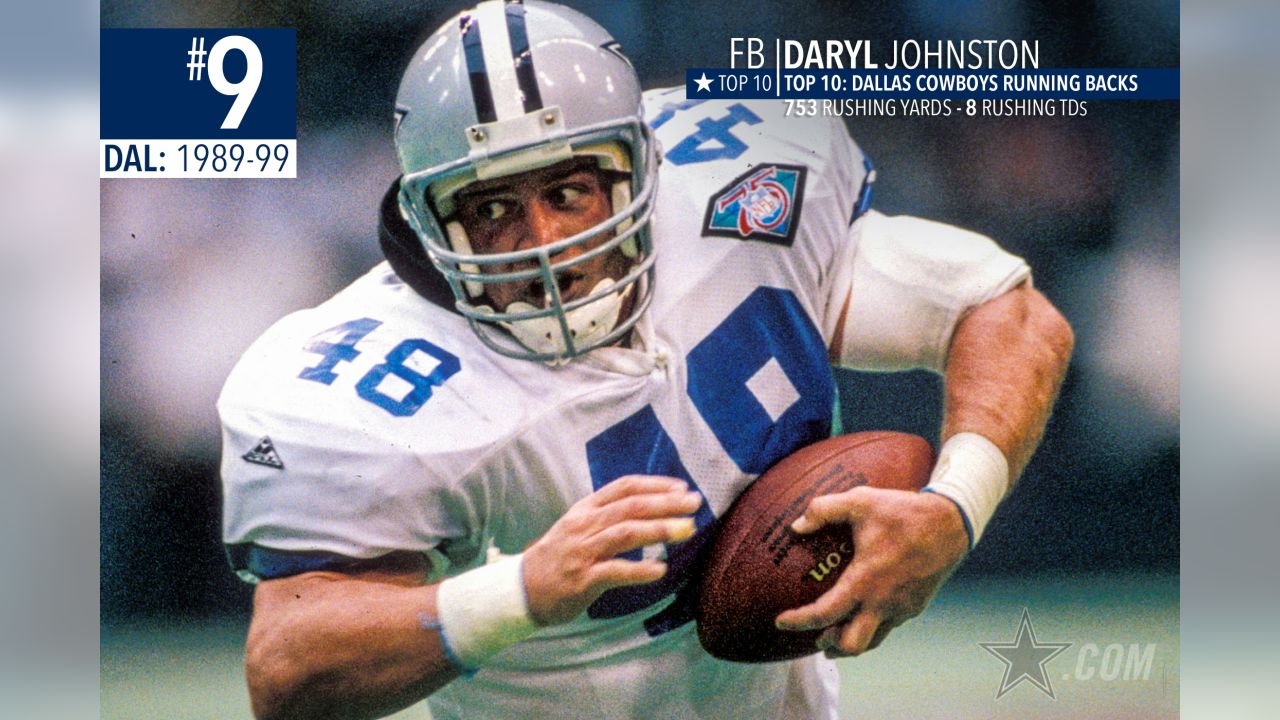The image is a horizontally aligned rectangle featuring Daryl Johnston, a prominent football player for the Dallas Cowboys. Johnston is centered in the frame, showcasing his athletic build and tan skin. He is donned in the iconic Dallas Cowboys white uniform with blue numbers, specifically number 48, which is visible on his shoulders and the front of his jersey. Johnston holds a football in his left hand and wears white wrist cuffs. His gray helmet features a distinctive navy and white stripe. With his mouth open, he appears to be in mid-action. 

The background has thick vertical borders blending gray and white shades. In the upper right corner, text reads: "FB/Daryl Johnston, Top 10 Dallas Cowboys running backs," followed by "753 rushing yards - 8 rushing TDs." A star symbol next to this text highlights his top 10 status. The upper left corner displays a large number 9 against a dark blue background with the text "DAL: 1989 to 1999" beneath it. The bottom right corner of the image includes a blue rectangle with a white star and "Star.com," indicating his ranking among the top 10 Dallas Cowboys running backs.